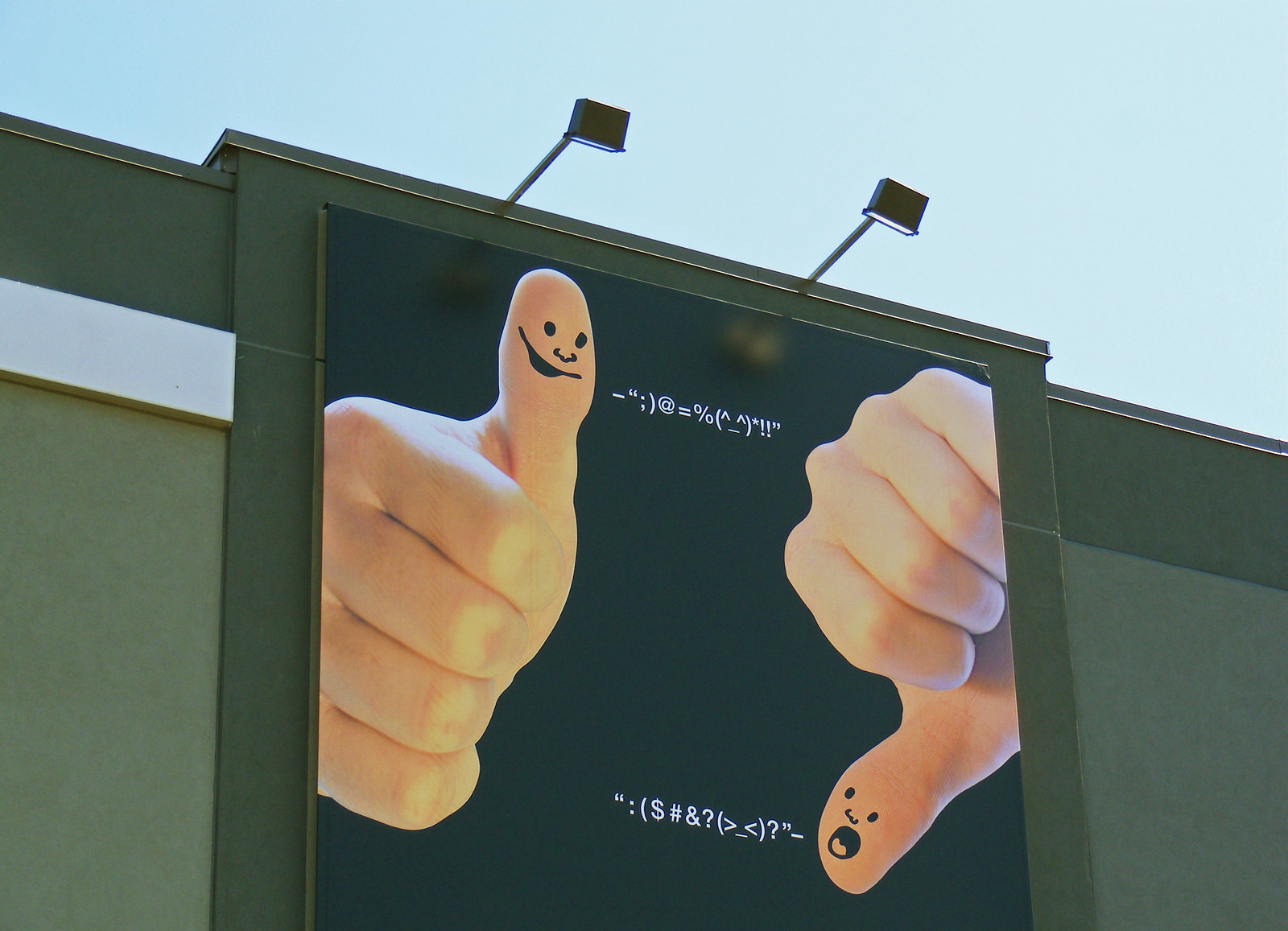In this image, a large billboard is prominently displayed on the side of a grayish building. The billboard is illuminated by two spotlights positioned at the top. The background of the billboard is black, highlighting the main elements in the foreground. Featured on the billboard are two hands: one giving a thumbs up and the other giving a thumbs down. Each thumb is adorned with a drawn face, adding a playful touch.

The thumb that is upright has a face with two eyes, a nose, and a mouth that is slightly open and positioned sideways, giving it a quirky expression. In contrast, the downward thumb sports a different set of facial features, with two eyes, a distinctively shaped nose, and a mouth that is round and dark inside, revealing a visible tongue. Equations emanate from the mouths of both thumbs, suggesting speech or thought bubbles.

To the left of the billboard is a white vertical strip, accentuating the borders of the billboard. The building itself features a grayish hue with a darker gray section at the top, adding a sense of depth and context to the urban setting.